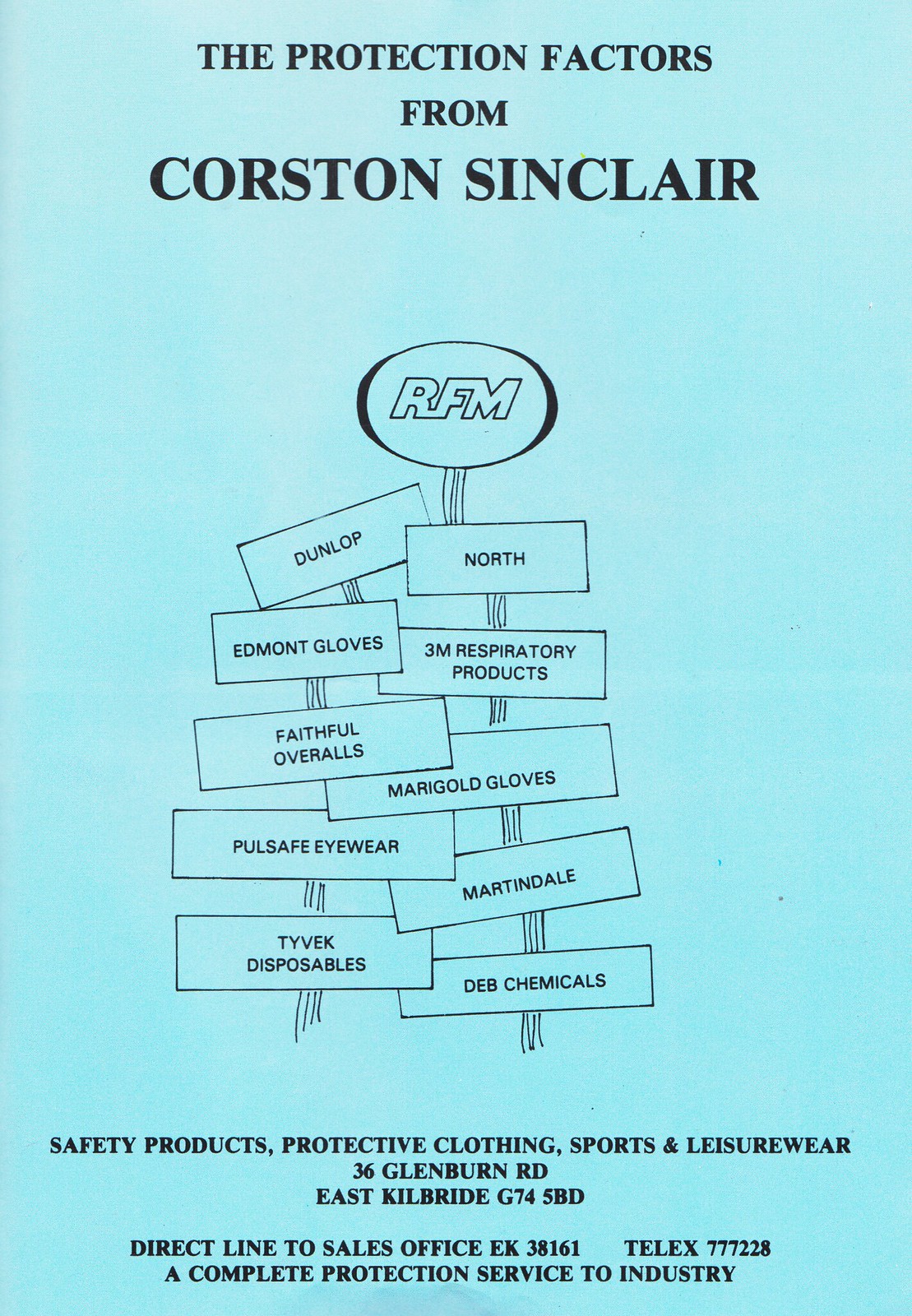The image is an advertisement poster with a light blue background and black, standard font. At the top, larger text reads "The Protection Factors from Korsten Sinclair." Below this heading, there is a central graphic resembling a wooden sign composed of various rectangles, each displaying different safety products and brands. 

At the apex of the graphic, an oval shape with the letters "RFM" stands out. Surrounding rectangles list the names Dunlop, North, Edmont Gloves, 3M Respiratory Products, Faithful Overalls, Marigold Gloves, PulseSafe Eyewear, Martindale, Tyvek Disposables, and DB Chemicals.

Towards the bottom, in bold lettering, the categories "Safety Products, Protective Clothing, Sports and Leisure Wear" are prominently displayed. The contact information includes the address "36 Glenburn Road, East Kilbride, G745BD," a direct line to the sales office at "EK 38161," and a Telex number "777-228." The tagline at the bottom reads, "A Complete Protection Service to Industry."